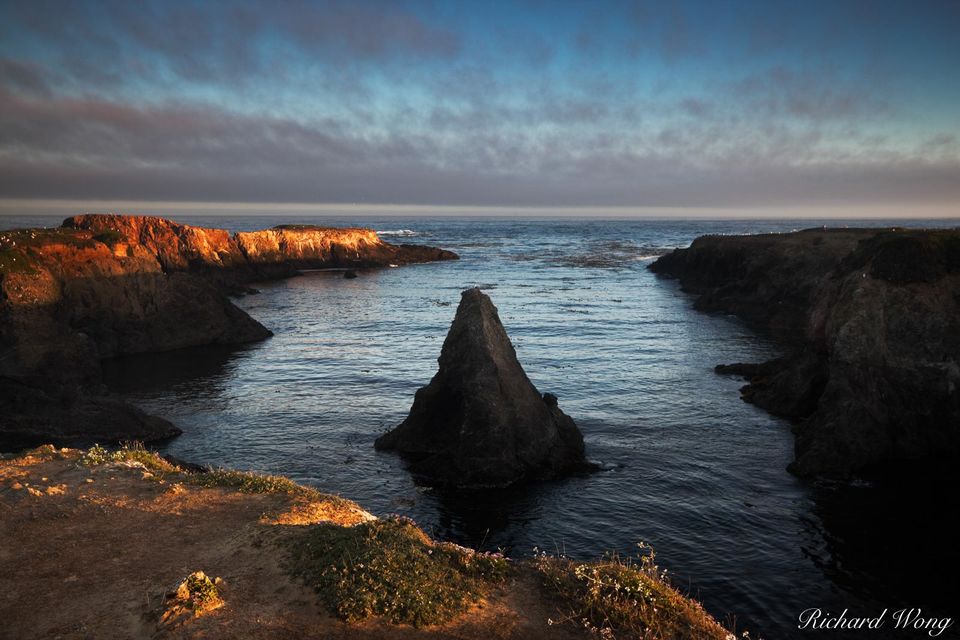This photograph, taken by Richard Wong at either sunrise or sunset, captures a dramatic coastal scene. Dominating the middle of the image is a rocky, pyramid-shaped outcrop, situated in a small bay that is surrounded by cliff faces and rocks. The outcrop, illuminated by a golden hue from the sun, adds an ethereal quality to the setting. The foreground features a sheer, rocky cliff where the photographer likely stood, adorned with patches of moss and small plants. To the left, the cliff faces are bathed in an orange glow, while the right side remains in shadow, enhancing the depth and contrast of the scene. The ocean is relatively calm within the bay, but in the distance, waves are breaking against the vast, open sea. Above, a sprinkling of thin clouds decorates an otherwise blue sky. The image also contains a subtle watermark with the photographer's name, Richard Wong, in cursive text. Redolent of rugged landscapes like those found in Scotland, the scene is both serene and majestic.